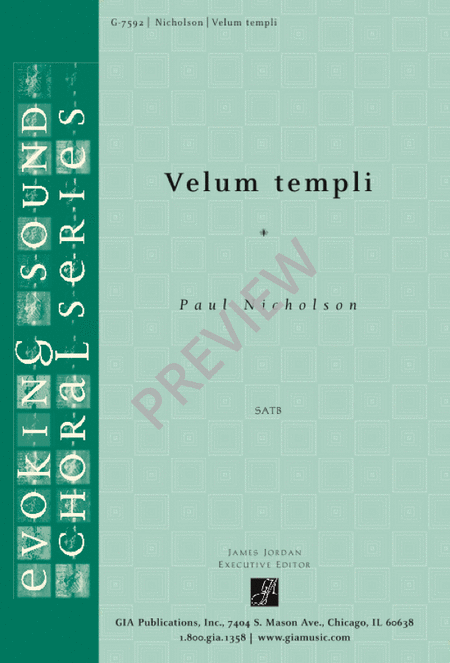The image features the cover of a music book titled "Vellum Templi" by Paul Nicholson. The background showcases different shades of green, with light green filling most of the area and darker green on the left side. Covering the entire background are square patterns that are a mix of light and dark grey, giving a faded appearance. The title "Vellum Templi" is prominently displayed at the top in black text, followed by the author's name, Paul Nicholson, also in black text at the center. A pink stamp marked "Preview" is tilted across the center of the cover. On the left side, in white font inside vertical boxes, is the text "Evoking Sound Choral Series." Additional details at the bottom provide the publisher's information: GIA Publications, Incorporated, located at 7404 South Mason Avenue, Chicago, IL 60638, along with a phone number, 1-800-GIA-1358, and the website www.giamusic.com. James Jordan is mentioned as the Executive Editor in the same section.